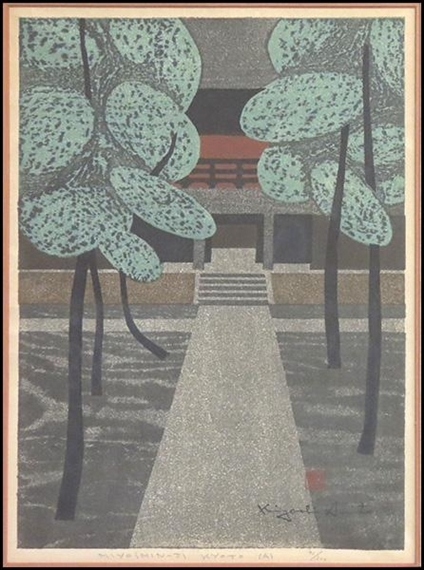The image is a vertical rectangular painting with a multi-layered frame: an outer thin black border, followed by a brown border, and a beige colored border inside. Central to the composition is a white gravel pathway, speckled with tiny white dots, cutting through the middle and leading to a set of four to five stone steps. These steps, equally speckled with white, ascend to another platform that appears to be part of a building. The building's entrance is an open square doorway, and above this entry is a second floor with a brown railing against a red backdrop, capped by a gray and black upper structure.

On both sides of the main pathway, there are darker gray sidewalks containing similar white specks. Flanking these sidewalks in the foreground is a mixed gray ground, featuring swirls of lighter gray tones. Trees are drawn on either side: three on the left and one or two on the right. These trees are depicted with thin black trunks and large oval leaves in light green, speckled with dark spots to suggest individual leaves.

The overall style suggests a combination of painting and drawing, characterized by an austere and somewhat stylized aesthetic. The scene is framed in a way that resembles a traditional painting, with contrasting frame colors enhancing its presentation.